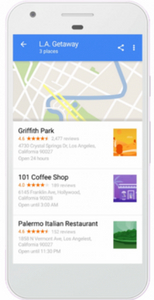The image depicts a smartphone screen showing a map and a collection of recommended destinations under the heading "LA Getaway." The top portion of the screen shows part of a map featuring a river, several roads, and two buttons: a share button and an ellipses menu button. Below the map, a blue box with the text "LA Getaway" is displayed prominently. The first recommendation listed is Griffith Park, which has a rating of four stars and a brief description underneath, accompanied by an orange and yellow thumbnail image. Following that, the 101 Coffee Shop is highlighted with a four-star rating, some descriptive text, and a purple thumbnail image. The final recommendation on the list is the Palermo Italian Restaurant, boasting a four and a half star rating, descriptive text, and a green thumbnail image. The overall quality of the image is blurry, making some of the text difficult to read.